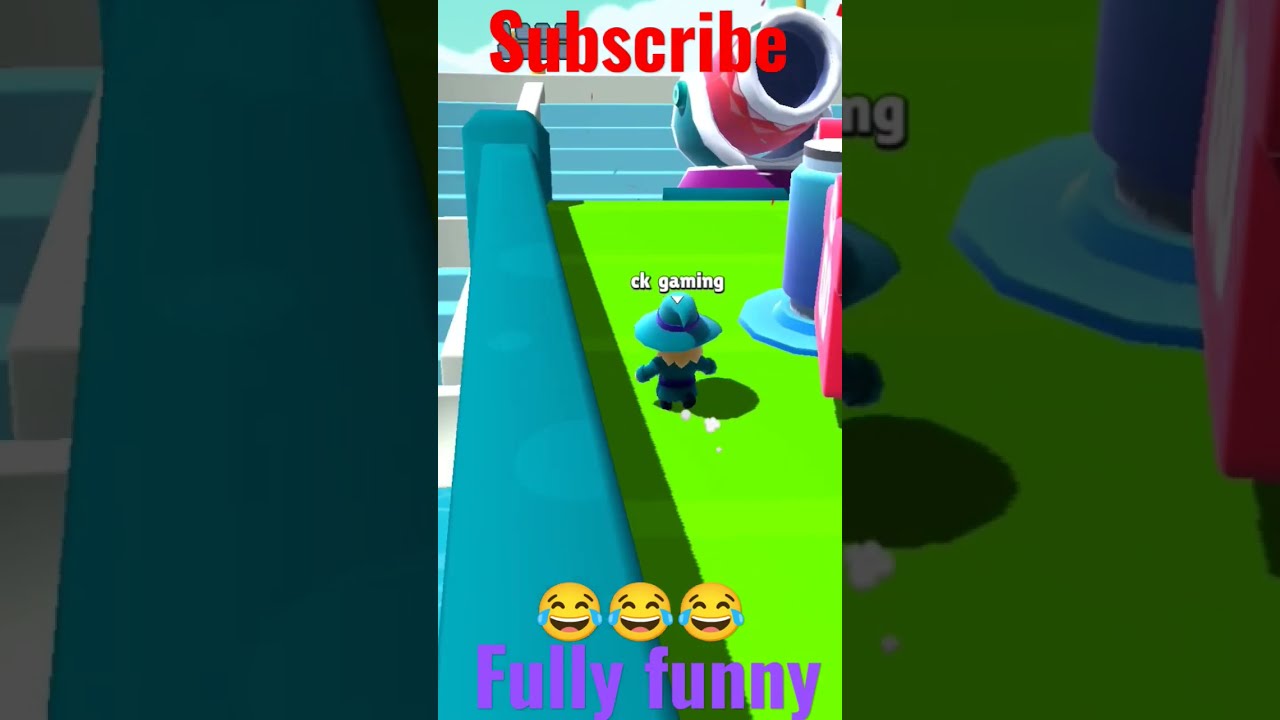This image depicts a vibrant, video game-themed channel banner. At the top in bold red letters is the word "Subscribe" with a capital 'S' and the rest in lowercase, urging viewers to follow the channel. Below, on a lush, bright neon green grassy backdrop, a character dressed in a vibrant teal witch's hat and matching outfit stands prominently. Above this character, "CK gaming" is written in small white letters on a black background. The character's ensemble includes a pointy teal hat, blue gloves, a blue belt, black boots, and they appear to be releasing puffs of white smoke behind them, casting a shadow over the green grass. In the scene is a blue racing track with light blue lines, white sidewalls, a blue sky with white clouds, and a large cannon in the top-right corner. At the bottom of the image, three emojis, laughing to the point of tears, decorate the scene, complemented by the words "Fully funny" in purple letters. The left side features a long blue pipe, amplifying the game's dynamic environment.